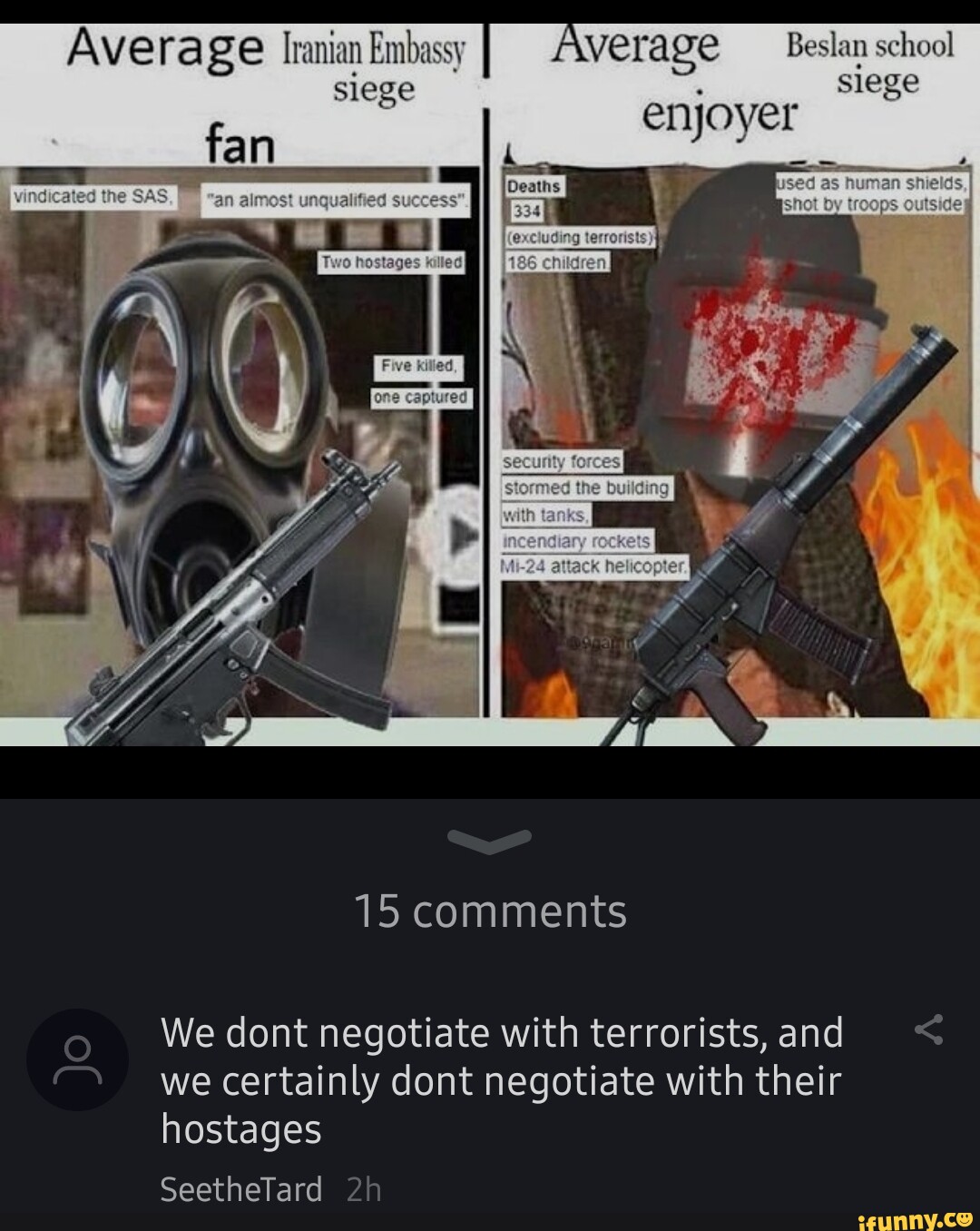Screenshot of a meme comparing the "Average Iranian Embassy Siege Fan" on the left to the "Average Beslan School Siege Enjoyer" on the right. The left side features a man in a gas mask holding a weapon, with multiple descriptive white boxes that include phrases like "vindicated the SAS" and "almost unqualified success". On the right, there is an image of a man in body armor, with blood on his face covering and holding a weapon. The meme has garnered interaction, with 15 comments in total and the top visible comment stating, "we don't negotiate with terrorists and we certainly don't negotiate with their hostages."